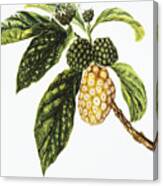This square photograph captures a botanical painting on a white canvas, slightly tilted to reveal its thickness. The main subject is a fruit-bearing tree branch that extends from the lower right to the upper left. The brown stem of the branch is visible on the front and side of the canvas. Prominently displayed in the composition is a large, yellow, pineapple-like fruit that resembles a cluster of circles. Above it, two green, berry-like fruits are positioned, along with healthy, oval-shaped green leaves. Further up the branch, additional leaves and another small berry sprout from the flowers. The artwork, rich in detail, portrays a vibrant and lifelike representation of the fruit and foliage against the stark white background, creating a vivid and realistic depiction.